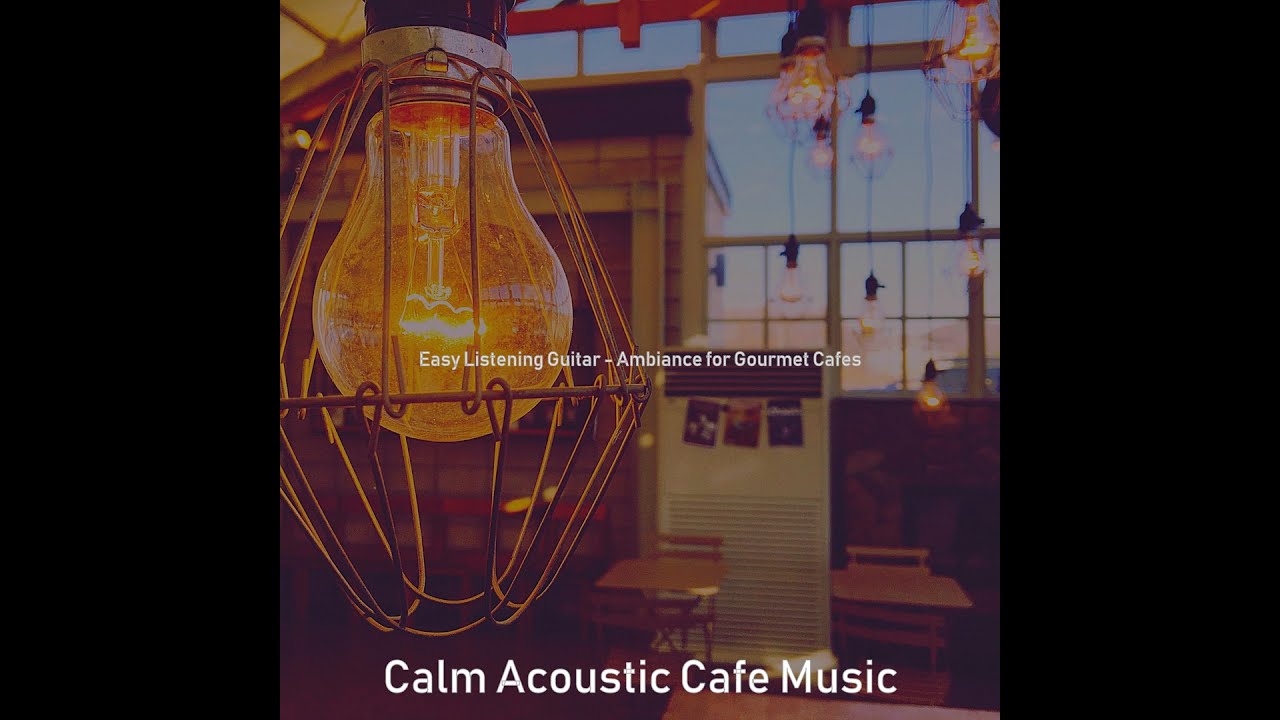The image, titled "Calm Acoustic Café Music," showcases a tranquil indoor café setting. Prominently on the left side of the image is a golden light bulb encased in a bronze, diamond-shaped frame. Several small wooden tables, each accompanied by two chairs, are scattered throughout the background. Behind one of these tables, a large window offers a view of a blue sky, suggesting it is daytime, potentially nearing sunset as it appears to be getting darker. From the ceiling in front of the window, numerous white light bulbs hang, adding a cozy ambiance to the café. The center of the image features text in white lettering stating "Easy-Listening Guitar Ambience for Gourmet Cafes," and at the bottom, similarly in white, it reads "Calm Acoustic Café Music." The overall palette includes black, yellow, orange, brown, red, silver, blue, and white, enhancing the warm and inviting atmosphere of the café.